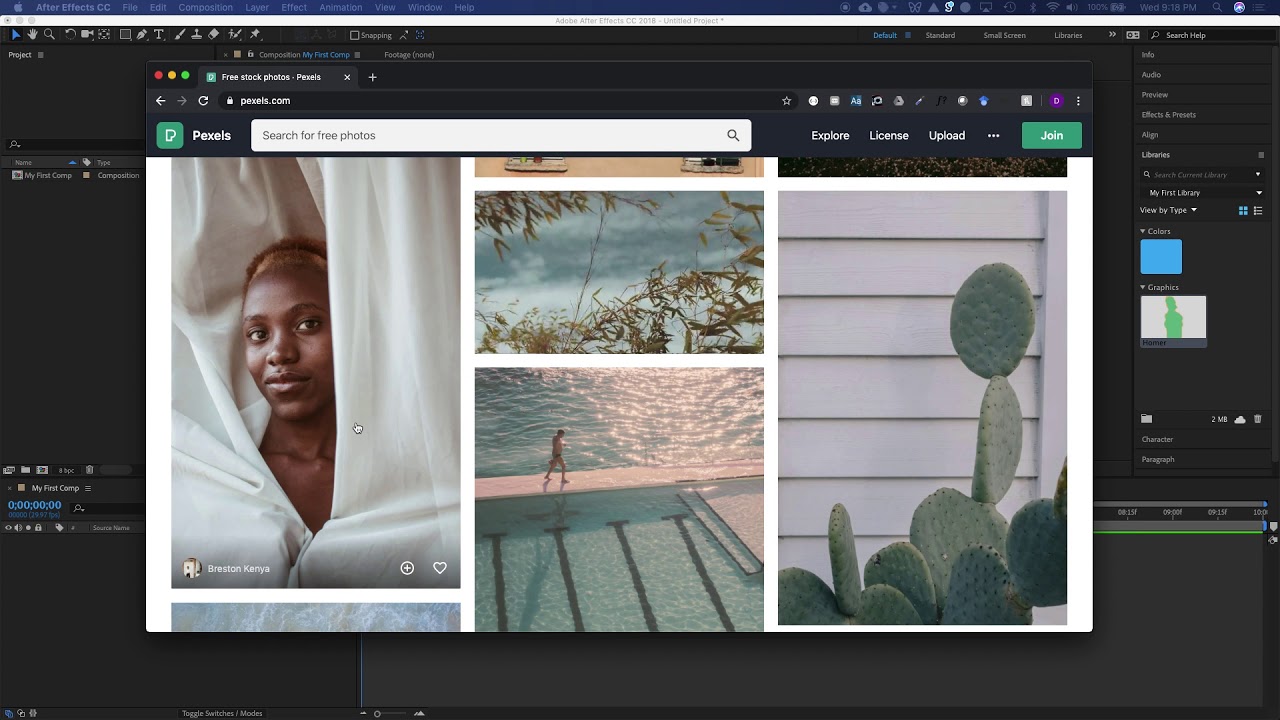Screenshot of a computer screen displaying an image search website. Across the top, there is a very thin, purplish bar with indiscernible elements due to its narrow size. Beneath the purple bar is a white bar that is largely nondescript. The primary focus of the screenshot is a black screen with numerous options displayed around it, though these options are partially obscured by a pop-up window.

The pop-up window features a green icon with the word "Pixels" and contains a search bar prompting users to "search for free photos," accompanied by a magnifying glass icon. To the right of the search bar, the black bar with white lettering includes the options: "Explore," "License," "Upload," and a menu represented by three dots for additional options. There's also a green "Join" button.

Beneath these elements, several photos are displayed, including:
1. A person peeking out from behind curtains.
2. Someone walking along a pool adjacent to a body of water.
3. A landscape view through trees.
4. A close-up of a cactus.

This setup suggests the diverse range of photos available for use on the platform.